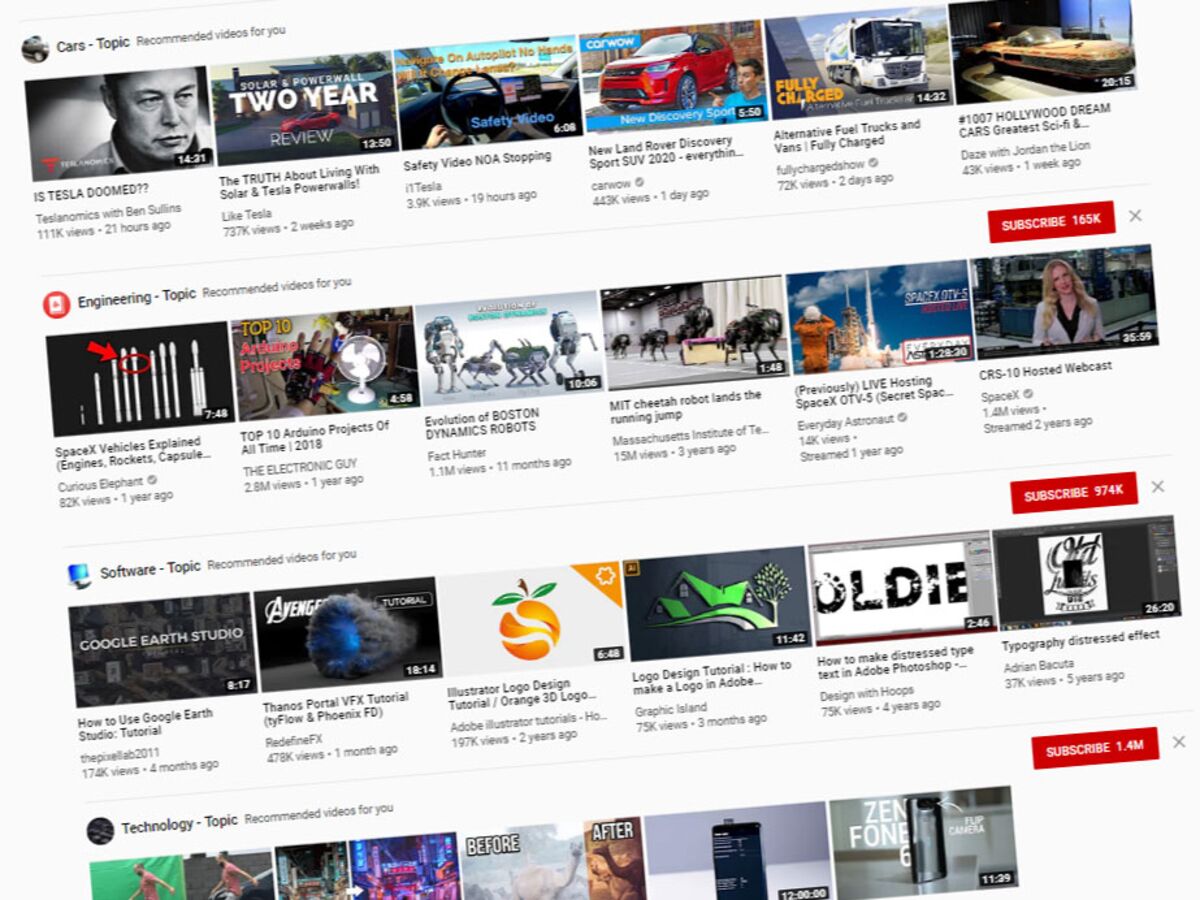The screen display showcases a variety of recommended video topics at an angled view. At the forefront is a prominent logo, and the content primarily revolves around cars and technology. The first row of videos includes titles such as:

1. "Is Tesla Doomed?"
2. "The Truth about Living with Solar and Tesla Powerwalls"
3. "Safety Videos: NOA Stopping"
4. "The New Land Rover Discovery Sport SUV 2020"
5. "Alternative Fuel Trucks and Vans"
6. "Fully Charged"
7. "Hollywood Dream Cars: Greatest Sci-Fi Vehicles"

The second row features videos under an "Engineering" topic, prompting viewers to subscribe for more content. Below this row are special sections explained, along with various technology-related articles. The lowest section on the screen delves into "Software Topics" and overlaps with general technology subjects. The displayed content suggests that the viewer is particularly interested in the latest updates and insights spanning from automotive innovations to cutting-edge technology and architectural designs.